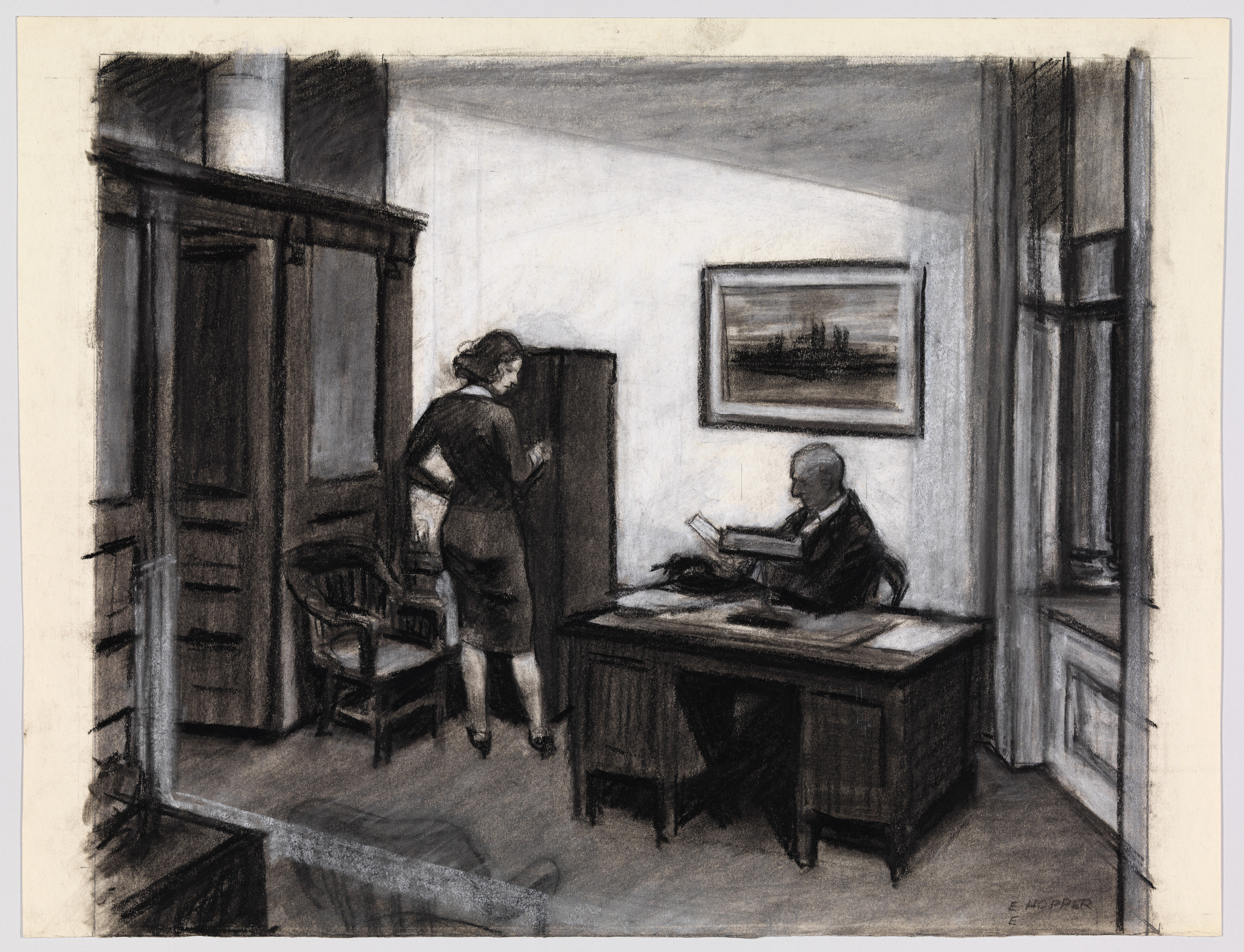A meticulously detailed, black and white charcoal drawing depicts a vintage office setting. At the center, a Caucasian man in a suit is seated behind an old-fashioned wooden desk, intensely focused on a piece of paper in his hand. His desk holds a classic landline telephone and a lamp, suggesting the scene likely takes place late in the day. Directly in front of him, a Caucasian woman, possibly his secretary, stands with her back to the viewer. She is dressed in a knee-length skirt and top, with dark hair styled appropriately for a bygone era. Her stance, hands on hips, suggests she might have just turned to address him or is preparing to leave the room. The compact office is further characterized by its old-fashioned furniture, including a wooden chair positioned behind the woman. To her right, there's a wall or half wall with a glass section, next to an open door. The background is filled with a mixture of windows and white walls adorned with a picture behind the man. The room features significant shading and detail, with lush textures indicating a dark exterior through the windows, contributing to the intriguing and historically rich atmosphere of the scene.